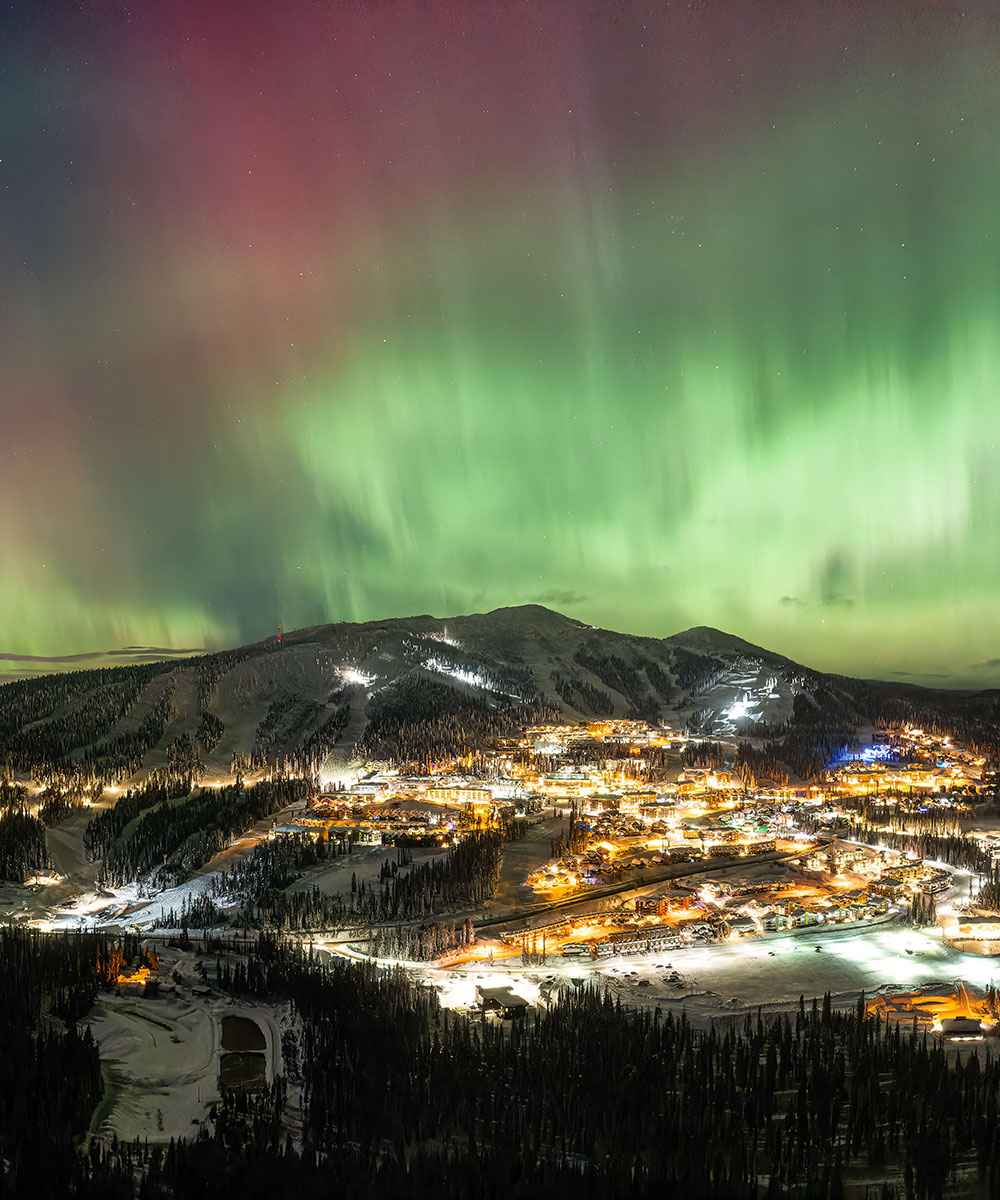The photograph captures a mesmerizing view of the Aurora Borealis, also known as the Northern Lights, enveloping a snowy arctic town under a sky aglow with vibrant greens, reds, and subtle touches of blue. This panoramic image reveals an overhead perspective of a well-lit, bustling valley populated with an array of buildings, lit streets, and numerous structures, giving the impression of a fully developed population center. Standing majestically in the background is a mountain range, its dark silhouette speckled with sparse patches of white snow. The vivid celestial display above saturates the entire scene in an unearthly light, while stars peek through the vibrant sky. Below this luminous spectacle, the town is abuzz with activity; you can discern parked cars, snowmobiles, and the tell-tale tracks of skiing enthusiasts crisscrossing the snow. The surrounding landscape features rows of evergreen trees and elevated terrain, creating a stark yet harmonious contrast to the illuminated townscape and the ethereal Aurora Borealis above.